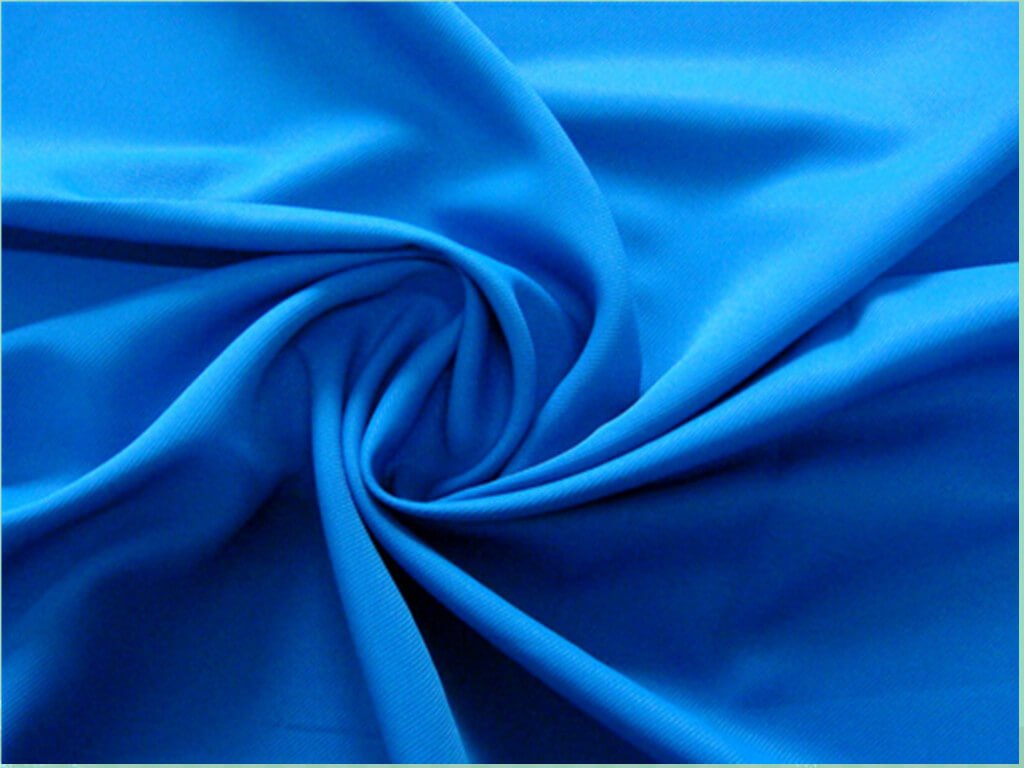This is a detailed photograph of a thick, royal blue fabric, meticulously swirled to create a captivating visual effect. The fabric, which could be similar to curtain or bedding material, is twisted from a central point, fanning out into fin-like folds. This technique, often achieved by using a fork to twist the material, results in an elegant and common presentation seen with items like restaurant napkins. The fabric dominates the entire image, free from any lettering or wording, allowing the intricate play of light and shadow to stand out. The folds, radiating towards the left, suggest the twist was made to the right. The light casts varying shades of blue across the surface—lighter shades appear on the top right, transitioning to darker hues towards the lower areas. Certain sections, especially near the twist's center, reveal deeper shadows, adding to the rich, textured appearance of the fabric.